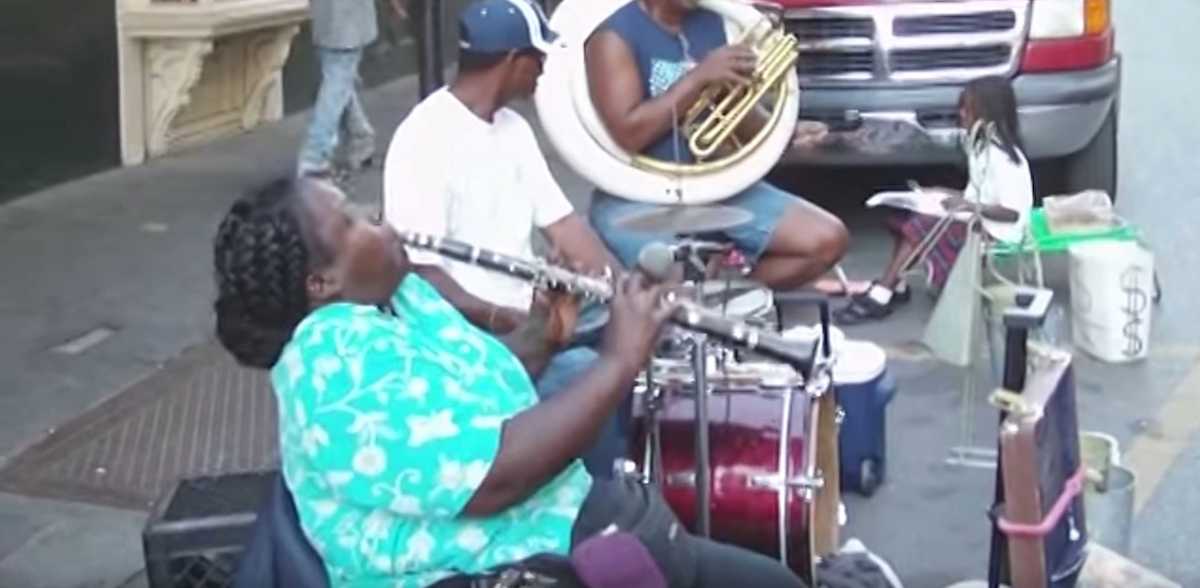The photograph captures a lively street performance taking place outdoors on a grey sidewalk, extending from the bottom left corner into the distance, marked by a rectangular, striated metal manhole cover. The primary focus is a group of street musicians who seem to be a family. They are positioned in front of a red Dodge pickup truck, with its lights on, adding a glow to the scene.

In the foreground, a soulful African American woman, adorned in a turquoise or blue button-down shirt with white floral designs, black pants, and black dreadlocks tied back, is passionately playing a clarinet. Her head is tilted back, immersed in the melody. To her immediate right, a man in a white t-shirt and jeans, possibly a drummer, sits beside a drum set, although he is not actively playing at the moment. He occupies a stool, casually observing the scene.

Further to the right, another man, dressed in a blue tank top and cutoff jeans, is handling a brass instrument—likely a tuba—with a smaller horn around his neck, positioning himself for the next tune. Beyond him, on the far right, a young girl in a plaid skirt, white shirt, white socks, and black shoes sits in a low chair close to the truck. She appears to be accepting donations, with a dollar-symbol bag next to her, and holding something indistinct on her lap, possibly a book or a small instrument. A weathered blue jeans-clad pedestrian walks along the grey sidewalk.

The photograph, with its slightly grainy texture, conveys a sense of community and shared joy among the musicians, who have gathered to entertain passersby and earn some donations. The casual arrangement of various chairs and containers around them adds to the informality and warmth of the street performance scene.